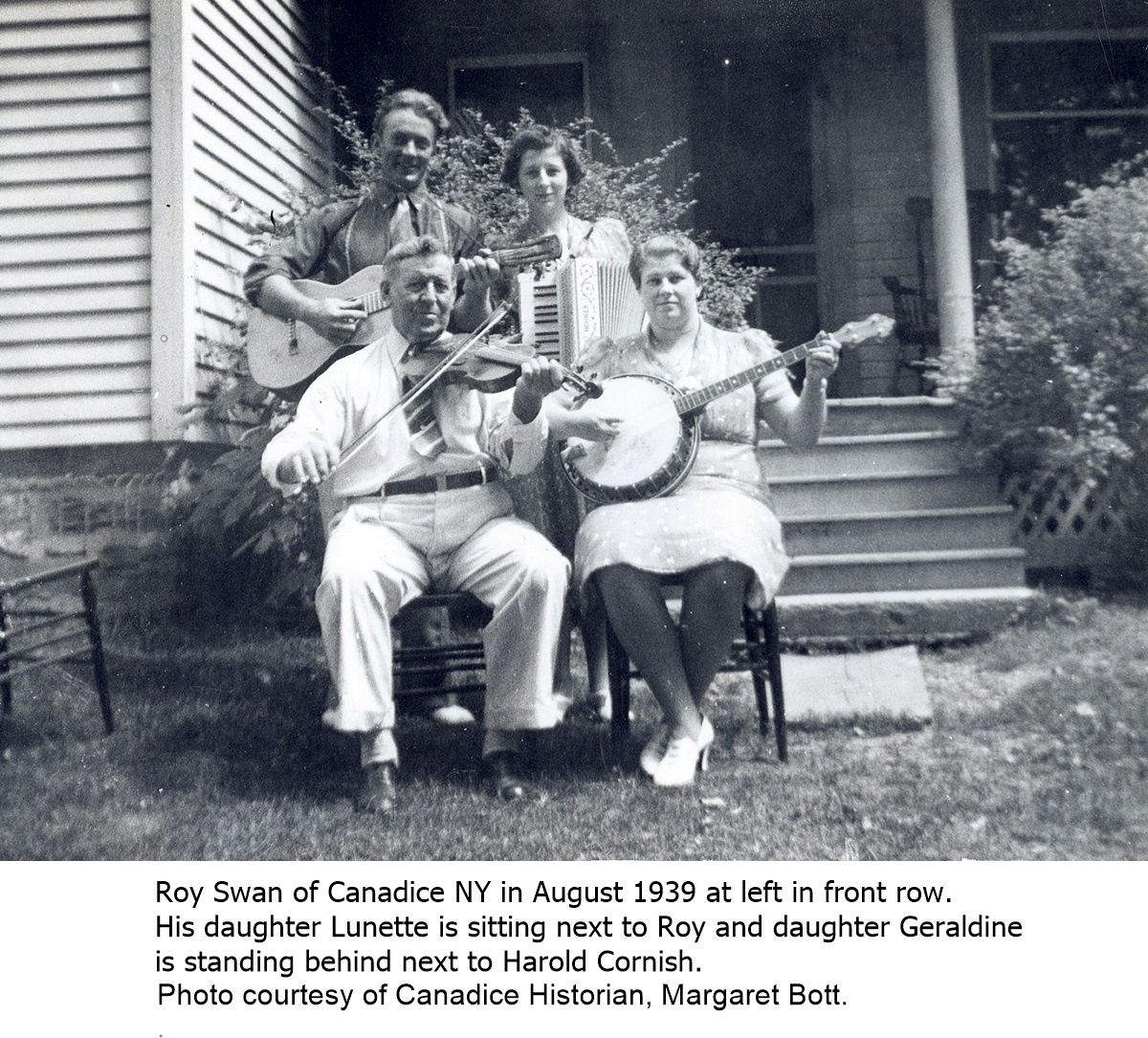This detailed black-and-white photograph depicts a musical family posing in front of a house with concrete steps and flanked by large bushes. Seated in chairs at the front are Roy Swan, holding a fiddle, and his daughter Lunette with a banjo. Standing behind them are Roy's daughter Geraldine, holding an accordion, and a younger man named Harold Cornish, pretending to play an acoustic guitar. The group looks happy and is positioned near an inviting front porch with a table and an empty chair to the left, suggesting a homely and musical atmosphere. To the right, there’s a tree adding to the scenic backdrop. The caption underneath reads, "Roy Swan of Kansas, New York, in August 1939, at left in front row. His daughter Lunette is sitting next to Roy and daughter Geraldine is standing behind, next to Harold Cornish. Photo courtesy of Canada's historian Margaret Bott."